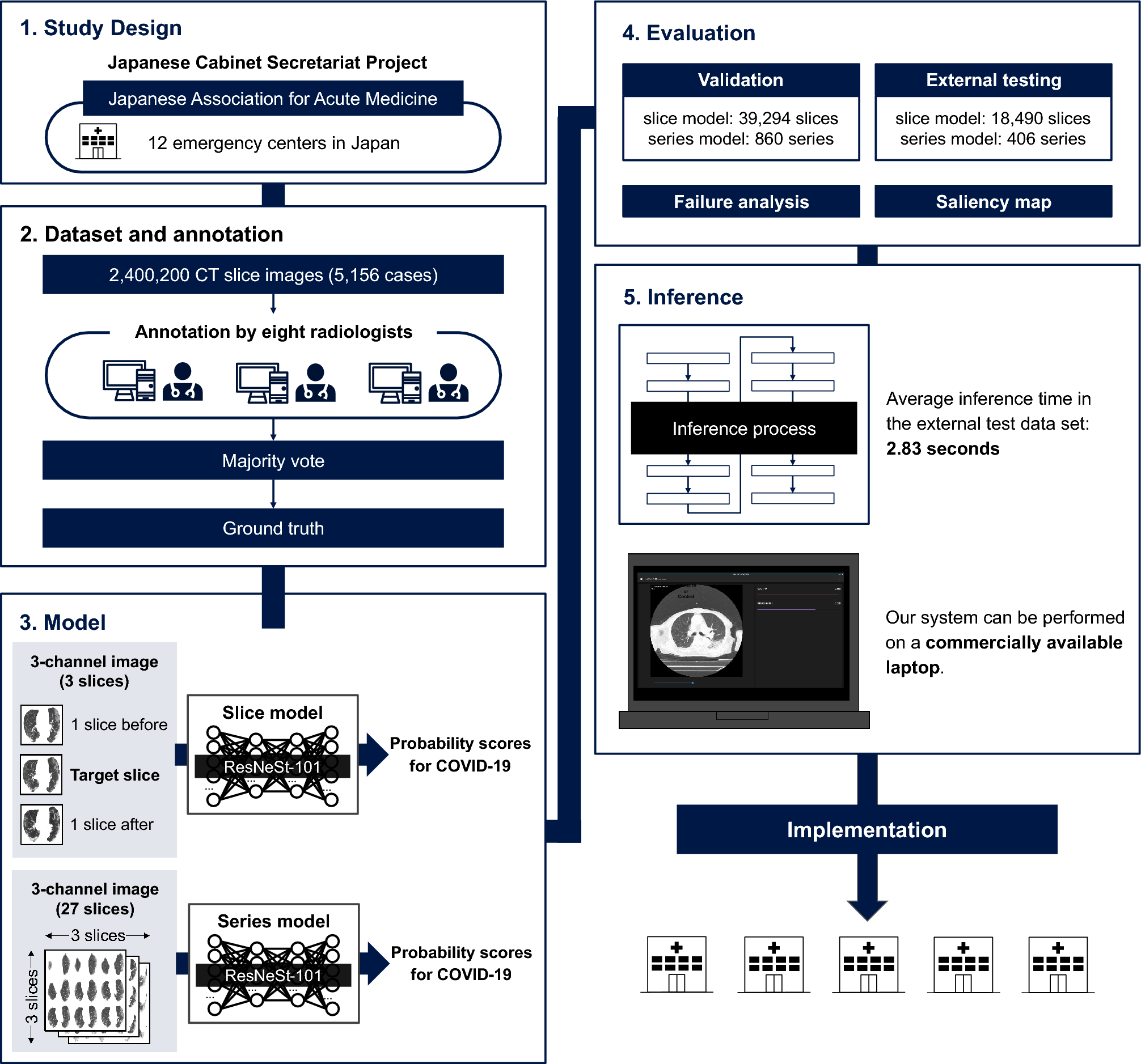The image is a detailed poster or slide from a presentation, likely aimed at depicting a Japanese medical protocol for evaluating and processing CAT-slice images, potentially in the context of COVID-19. The left page, numbered 1-3, introduces the "Study Design" involving the Japanese Cabinet Secretariat Project, the Japanese Association of Acute Medicine, and 12 emergency centers in Japan. It further explains that the "Data Set and Annotation" includes 24,400 CAT-slice images from 5,156 cases. Accompanying this is a diagram showing a person standing next to a computer screen, indicating an educational or instructional context akin to a PowerPoint presentation. The "Model" section lists various imaging techniques, such as MRI and CAT scans. The right page, numbered 4-5, delves into "Evaluation," breaking it down into "Validation," "External Testing," "Failure Analysis," and "Saliency Map." The "Inference" section outlines the inference process, noting that the system operates on commercially available laptops. Below this, an "Implementation" section features five hospital buildings, illustrating the practical application of the system in hospital settings. The flowchart effectively details how Japanese medical facilities acquire, process, evaluate, and implement radiological data to manage public health concerns, prominently illustrating a structured response protocol potentially tailored for the COVID-19 pandemic.